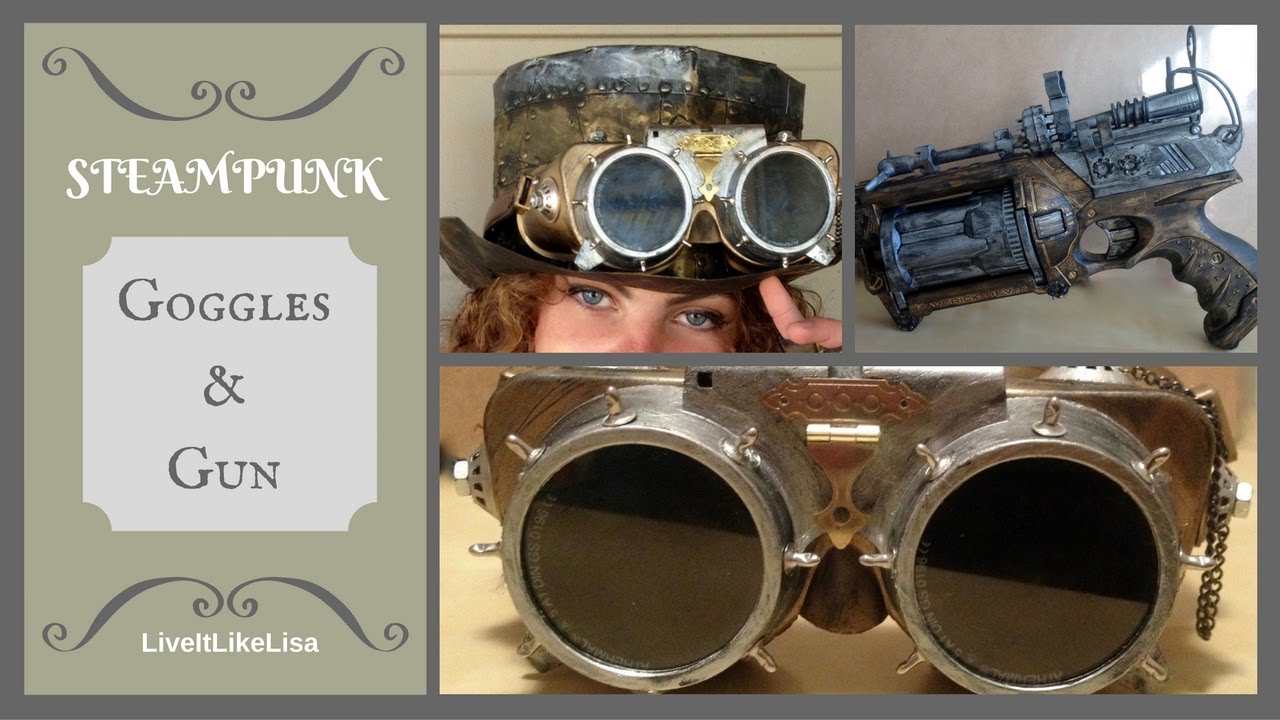This steampunk-themed image features various elements of the genre, prominently displaying the text "Steampunk" in a white serif font on the left side, along with "Goggles and Gun" in a dark gray serif font against a light gray background. At the bottom, the phrase "Live it like Lisa" is also visible in white text.

On the right side, the image is divided into sections. At the top left of this section, there's a close-up of a woman with vibrant blue eyes and curly, brownish-blond hair. She wears a distinctive, tall, riveted metal hat with a thin round brim, which also features a pair of silver goggles adorned with metal studs and brass-colored plating around the eyepieces.

Below this, there's another picture focusing on the same pair of steampunk goggles, emphasizing the intricate details of their design, including the black circles with silver rings and the brass-colored backing.

To the upper right, the image shows a steampunk revolver-style gun, featuring a revolving barrel, silver tubing on the upper part, and a handle at the back. The gun is ornately detailed with brass-colored trim, embodying a blend of futuristic and retro aesthetics reminiscent of the Borderlands video game series.